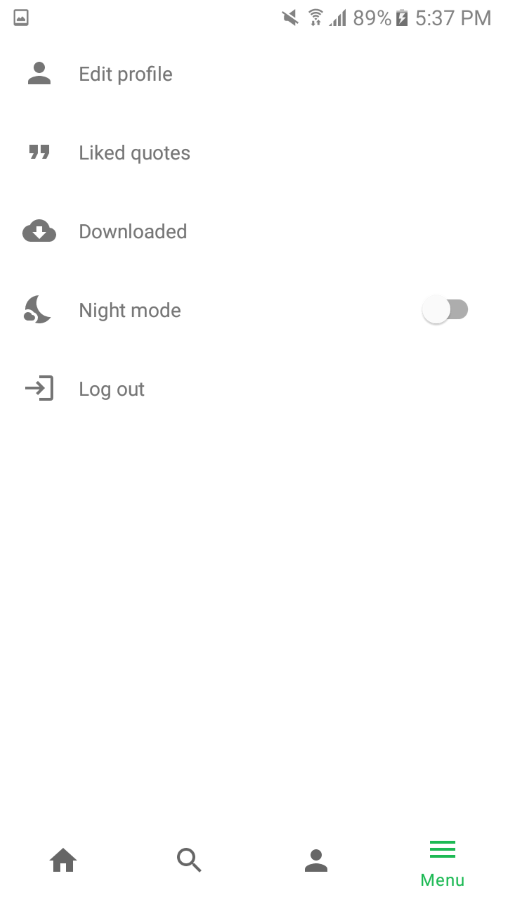The screenshot displays a phone app interface with a white background. At the top left corner, there are icons indicating a phone signal, Wi-Fi signal, and network strength. On the right side of the top bar, battery life shows at 89%, and the time is 5:37 p.m. Below the top bar, the screen features several menu options, including "Edit Profile," "Night Mode," and "Log Out." The "Night Mode" option is toggled on, indicated by a sliding button. At the bottom of the screen, there are navigation icons for Home, Search, and another icon that resembles a cat. Additionally, there is a menu represented by three horizontal lines, which is highlighted in gray. Each tab and button is accompanied by small icons that align with their respective functions. The overall design maintains a clean, minimalist layout with gray and white tones.